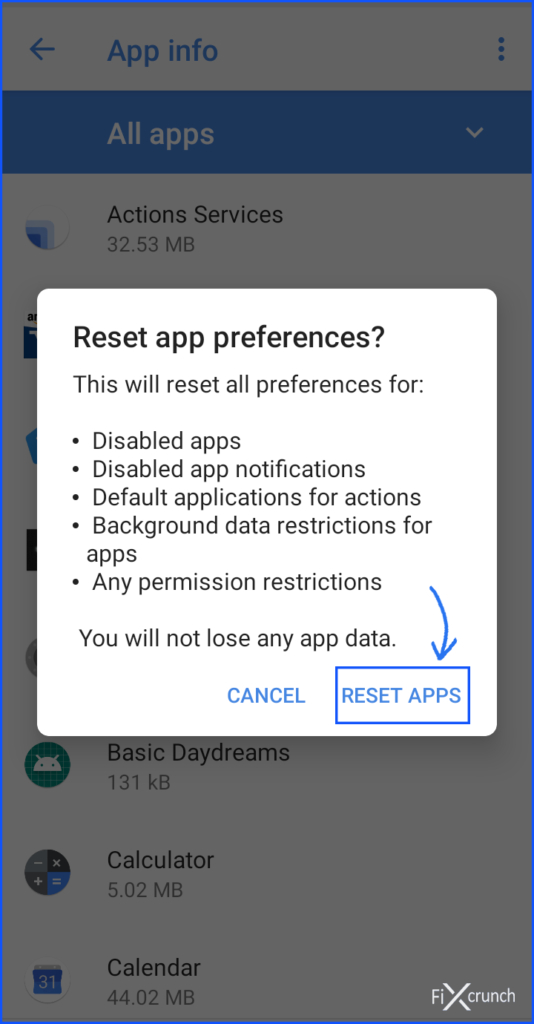This image appears to be a screenshot from a mobile application's "App Info" page. At the top of the screen, there is a white border with the title "App Info" displayed in blue text. Below this, a blue-bordered rectangular section labeled "All Apps" is visible against a white background. 

The main content of the page is a list of applications along with their respective icons and sizes. The first item listed is "Action Services" which occupies 32.53 MB of storage. Its icon features a circle with a blue corner. Next is "Basic Daydreams," at 131 KB, represented by a green circle with a white alien head icon. The third item, "Calculator," occupies 5.02 MB and is represented by an icon featuring mathematical symbols. This is followed by "Calendar," which uses 44.02 MB and is symbolized by an icon with the number "31" on a blue calendar page.

A white rectangular pop-up window partially covers the list, dimming the background. This pop-up is labeled "Reset App Preferences" in black text, and contains a brief description explaining the reset action: "This will reset all preferences for:" followed by a bullet list detailing what will be reset, including Disabled Apps, Disabled App Notifications, Default Applications for Actions, Background Data Restrictions for Apps, and Any Permission Restrictions. The message concludes with the note, "You will not lose any app data."

At the bottom of this pop-up, there are two blue text links: "Cancel" on the left and "Reset Apps" on the right. The "Reset Apps" link is highlighted with a blue rectangle outline, and an accompanying blue arrow points to it, indicating it as a selectable option.